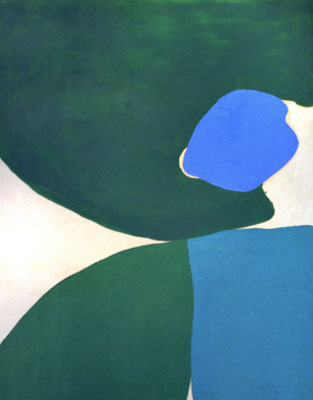This abstract painting features a predominantly dark green upper half, resembling a wave pattern that's mirrored, with its crest at the bottom. This dark green extends to a small part at the bottom left of the canvas, connecting with other sections. In the middle of the upper right quadrant, there's a circular splotch of sky blue surrounded by a white frame. The bottom right quadrant is dominated by a turquoise rectangle, which has irregular sides, and next to it on the left is a dark green shape resembling a leaf. The remaining areas of the painting are filled with white, including a triangular white shape in the bottom left quadrant and a squiggly white area in the middle. The overall composition is a blend of dark green, blue, and white colors arranged in an intriguing, seemingly random manner. The painting is a vertical rectangle.